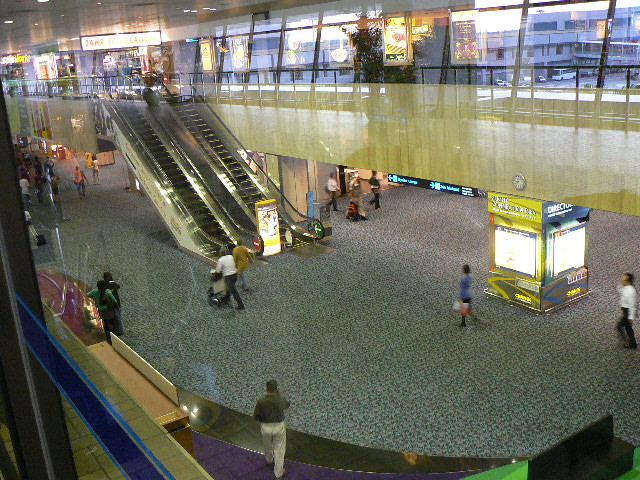The image captures a bustling interior scene of an airport, possibly a bit dated due to slight pixelation. It is taken from the second floor and showcases a spacious, open area. On the left side of the photo, there are two escalators, one leading upstairs and the other downstairs. Multiple people are visible: a man in a green shirt on his phone and another in a white shirt also conversing via cell phone. A person is seen pushing a luggage cart. The glass wall with railings offers views of the outside, revealing parked buses and cars, indicating it's daytime. There are several storefronts and restaurants on the second floor, their lights and signs reflecting off surfaces. Additional details include a directional wave sign on the bottom floor pointing towards the escalators and various kiosks and advertising billboards with illuminated screens dispersed throughout, adding to the busyness of the scene.